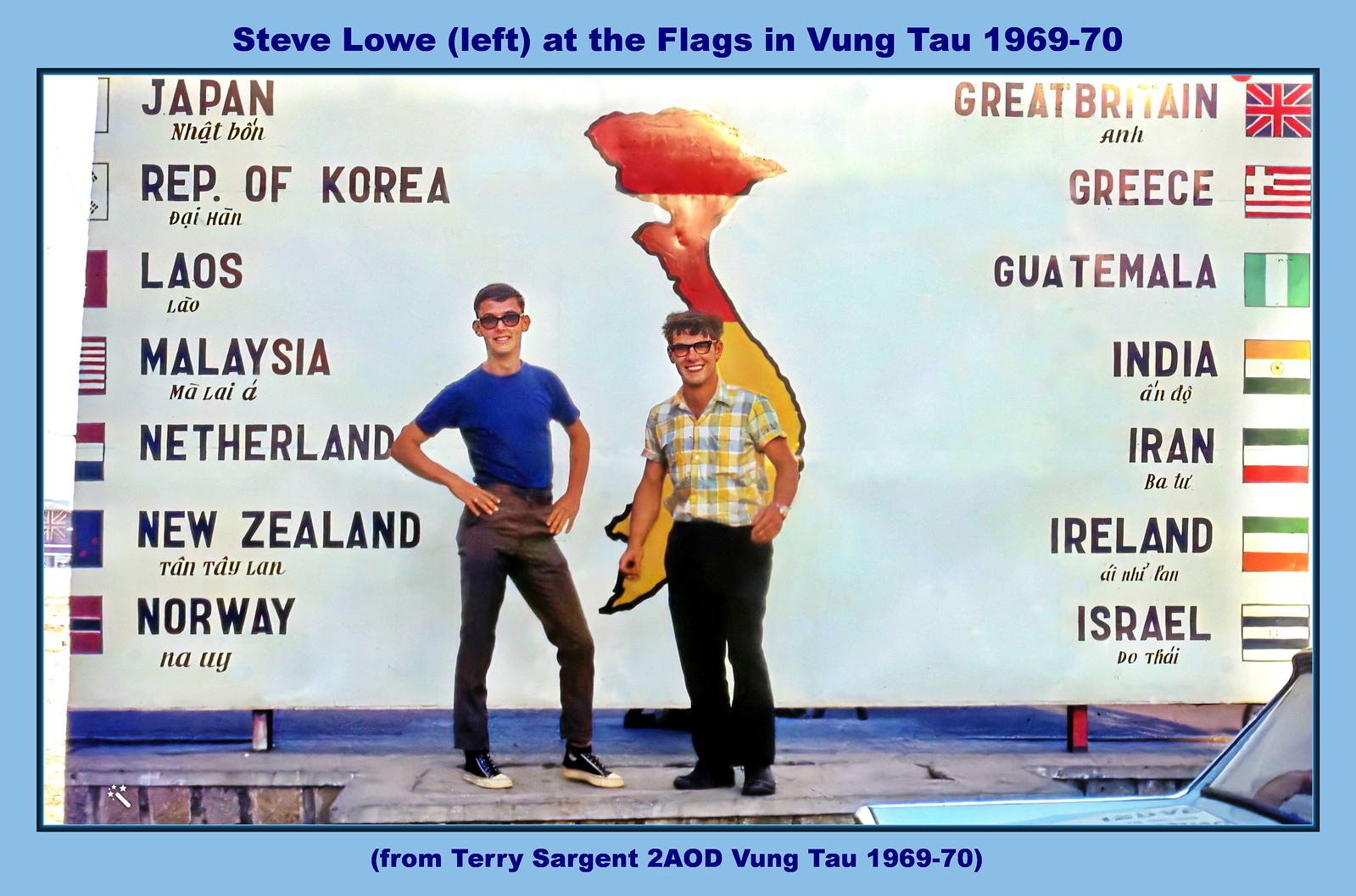The image captures two men standing on a stage-like platform, both wearing glasses and posing for the camera. The man on the left is dressed in a blue t-shirt, dark gray pants, and Converse-style sneakers, while the man on the right, who is shorter, sports a white, blue, and yellow striped short-sleeved shirt, black pants, dress shoes, and a watch on his left wrist. Behind them is a backdrop featuring a red and yellow map of Vietnam and an array of international flags, representing countries such as Japan, the Republic of Korea, Laos, Malaysia, the Netherlands, New Zealand, Norway, Great Britain, Greece, Guatemala, India, Iran, Ireland, and Israel. The display includes text at the top stating, "Steve Lowe left at the flags in Vung Tau 1969-1970," and at the bottom, it reads, "From Terry Sergeant to AOD Vung Tau 1969-1970."